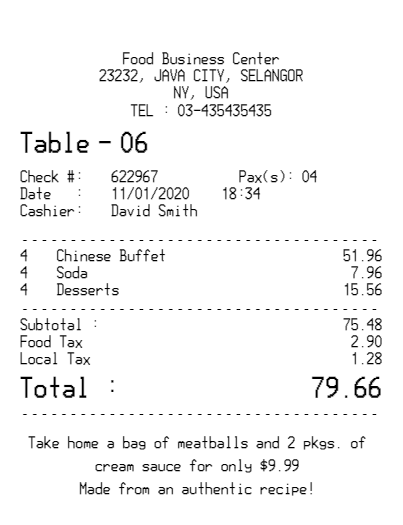This image displays a detailed restaurant receipt with black lettering on a white backdrop. At the top, the receipt features the name of the establishment: Food Business Center, located at 23232 Java City, Selangor, with an additional reference to New York, USA. The contact number listed is 03-435 435 435. Information on the left includes the table number (Table-06), check number (#622967), and the date of service (November 1, 2020), along with the cashier's name, David Smith. The items ordered consist of four Chinese buffets totaling $51.96, four sodas at $7.96, and four desserts amounting to $15.56. The subtotal comes to $75.48, with a food tax of $2.90 and local tax of $1.28, culminating in a total of $79.66. Additionally, the receipt mentions a take-home offer of a bag of meatballs and two packages of cream sauce for $9.99, touted as being made from an authentic recipe.